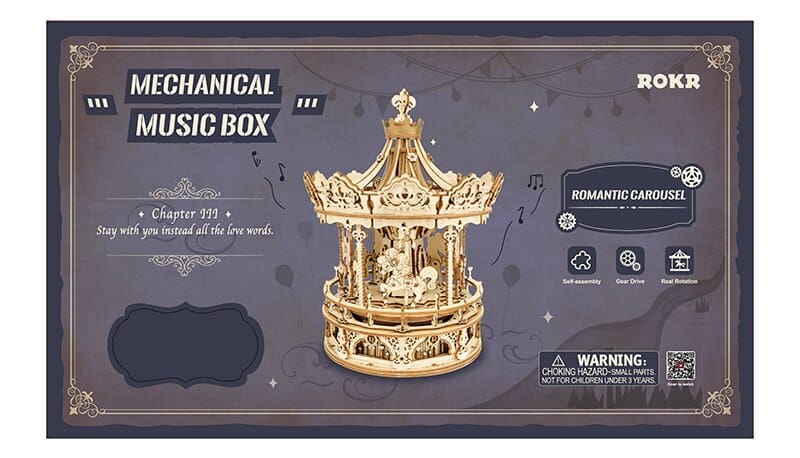This image is a detailed close-up of the packaging for a product called the "Mechanical Music Box" by ROKR. The central focus is a miniature, old-fashioned carousel with intricate horses and pillars, suggesting a whimsical, romantic theme. The main text in the upper left corner reads "Mechanical Music Box, chapter 111: Stay with you instead, all the love words." The right side features several key product descriptions within a dark gray square with rounded corners, including "romantic carousel," "self-assembly," "gear drive," and "real rotation," each accompanied by icons like gears, a puzzle piece, and a musical note. Below these descriptions is a cautionary warning: "Choking hazard, small parts, not for children under 3 years old," along with a QR code. The background features shades of gray and gold, with additional decorative elements such as balloons, musical notes, and streamers hanging overhead. An audible emphasis is placed on the carousel prominently situated in the center, sitting as if on the edge of a table. The entire design is framed by a gold border, enhancing its elegant and vintage appearance.